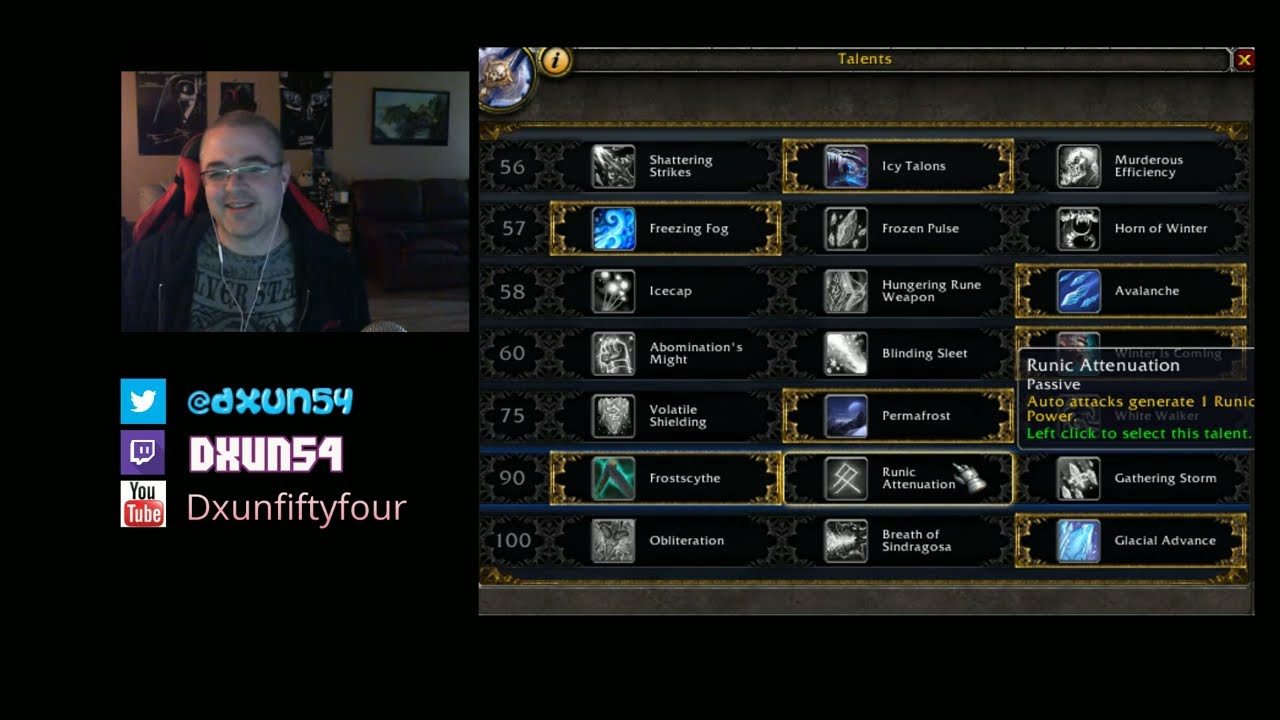This image depicts a male streamer, identifiable by his Twitter handle "@DXUN54," wearing glasses and wired earbuds, sitting in a red gaming chair in what appears to be his living room, evidenced by a black leather couch and pictures on the wall. His YouTube handle, "DXUNFIFTYFOUR," is also displayed. He is playing a game, the on-screen interface of which occupies the right side of the image. The interface is centered around the "Talents" menu, showing a grid of talent options, some of which are highlighted with a gold trim. The talents displayed include Shattering Strikes, Icy Talons, Murderous Efficiency, Freezing Fog, Frozen Pulse, Horn of Winter, Ice Cap, Hungering Rune Weapon, Avalanche, Abomination's Might, Blinding Sleet, Runic Attenuation, Volatile Shielding, Permafrost, Frost Scythe, Gathering Storm, Breath of Sindragosa, Obliteration, and Glacial Advance. A notable talent option, "Runic Attenuation - Passive: Auto Attacks Generate One Runic Power," indicates it can be selected by a left-click.